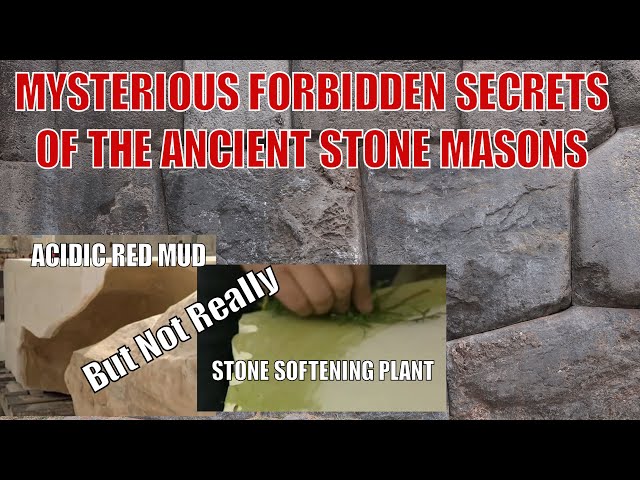The image features a backdrop of assorted grey stone tiles. Across the top, in bold, all-caps red letters with a white border, is the title: "MYSTERIOUS FORBIDDEN SECRETS OF THE ANCIENT STONE MASONS." At the bottom left is a box containing the bold text "ACIDIC RED MUD," also in white letters. To its immediate right is another box labeled "STONE SOFTENING PLANT," showing a man's hand applying a green plant to the stones. Diagonally across both boxes is the phrase "BUT NOT REALLY," suggesting a dubious claim about the plant's ability to soften stone. The image appears to depict a still from a video exploring mysterious and perhaps fictional practices attributed to ancient stonemasons.